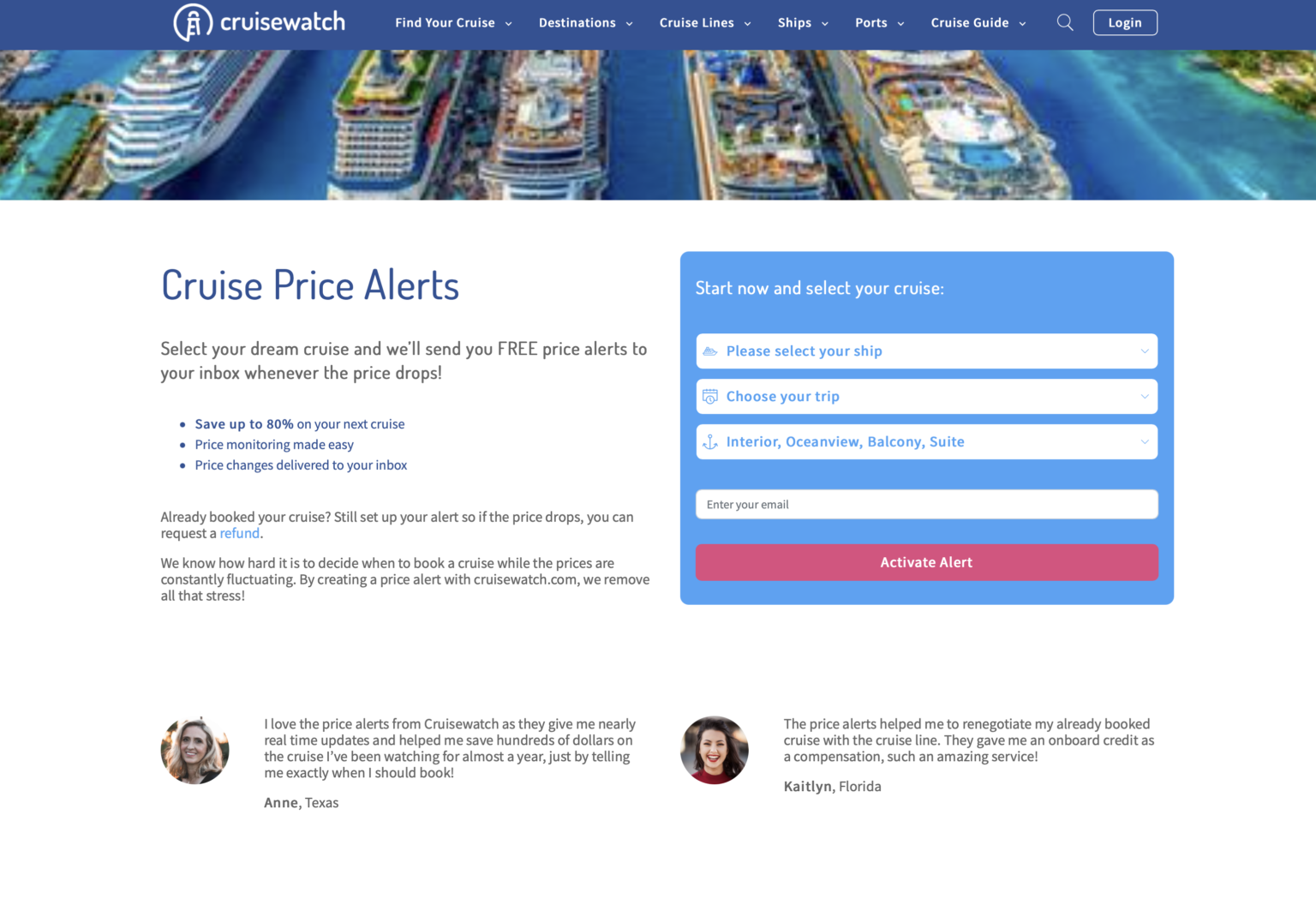This is a detailed screenshot of the CruiseWatch website. At the top of the page, a long horizontal blue banner stretches across the screen. On the left side of the banner, a logo featuring a lighthouse centered within a white circle is displayed, with the website name "CruiseWatch" written to its right. The navigation menu includes options labeled "Find Your Cruise," "Destination," "Cruise Lines," "Ships," "Ports," "Cruise Guide," "Search," and "Log In."

Just below this menu bar, there is a wide, horizontal aerial photograph capturing five cruise ships docked in tranquil blue waters. The image provides a top-down perspective, emphasizing the grand scale and arrangement of the vessels.

Below the image, text reads: "Cruise Price Alerts. Select your dream cruise and we'll send you free price alerts to your inbox whenever the price drops. Save up to 80% on your next cruise. Price monitoring made easy. Price changes delivered to your inbox." Next to this text, on the right, is a blue box where users can interact with the site. This box allows users to select specific details for their trip such as the ship, trip details, and room style (options include interior, ocean view, balcony, or suite). Additionally, users can enter their email address in this section to activate the price alert feature.